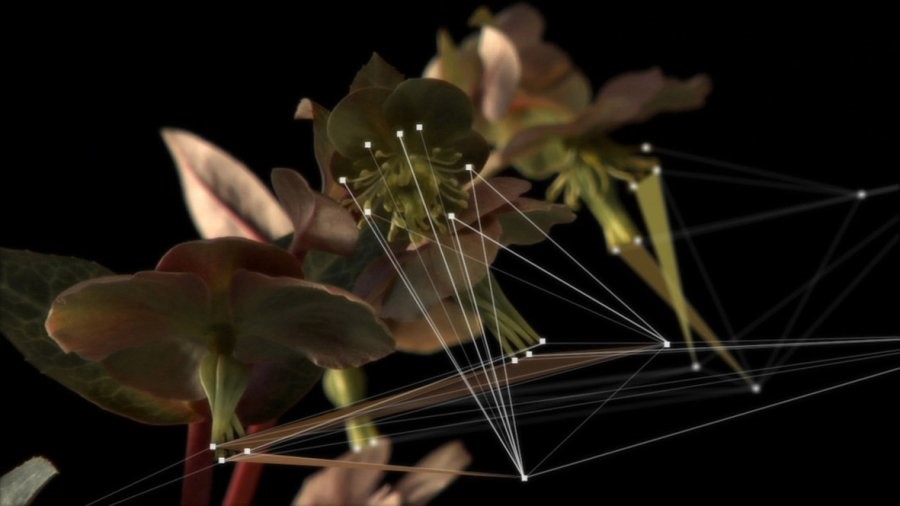This image captures a vibrant and detailed close-up of a plant with green leaves and orchid-like flowers in shades of red and light salmon. The plant is set against a stark black background, making its colors stand out vividly. Superimposed on this photograph is a complex network of white lines and small white dots, creating intricate patterns reminiscent of vector art. These lines crisscross the plant, converging at various points and forming triangular shapes with colors sampled from the plant, such as green and brown. The floral elements like pistils and stamens, though slightly out of focus, lead the viewer's eye from the lower left to the top center of the image. The pattern of lines is densely concentrated towards the bottom half and in the center, adding both a dynamic and organized layer to the botanical subject.